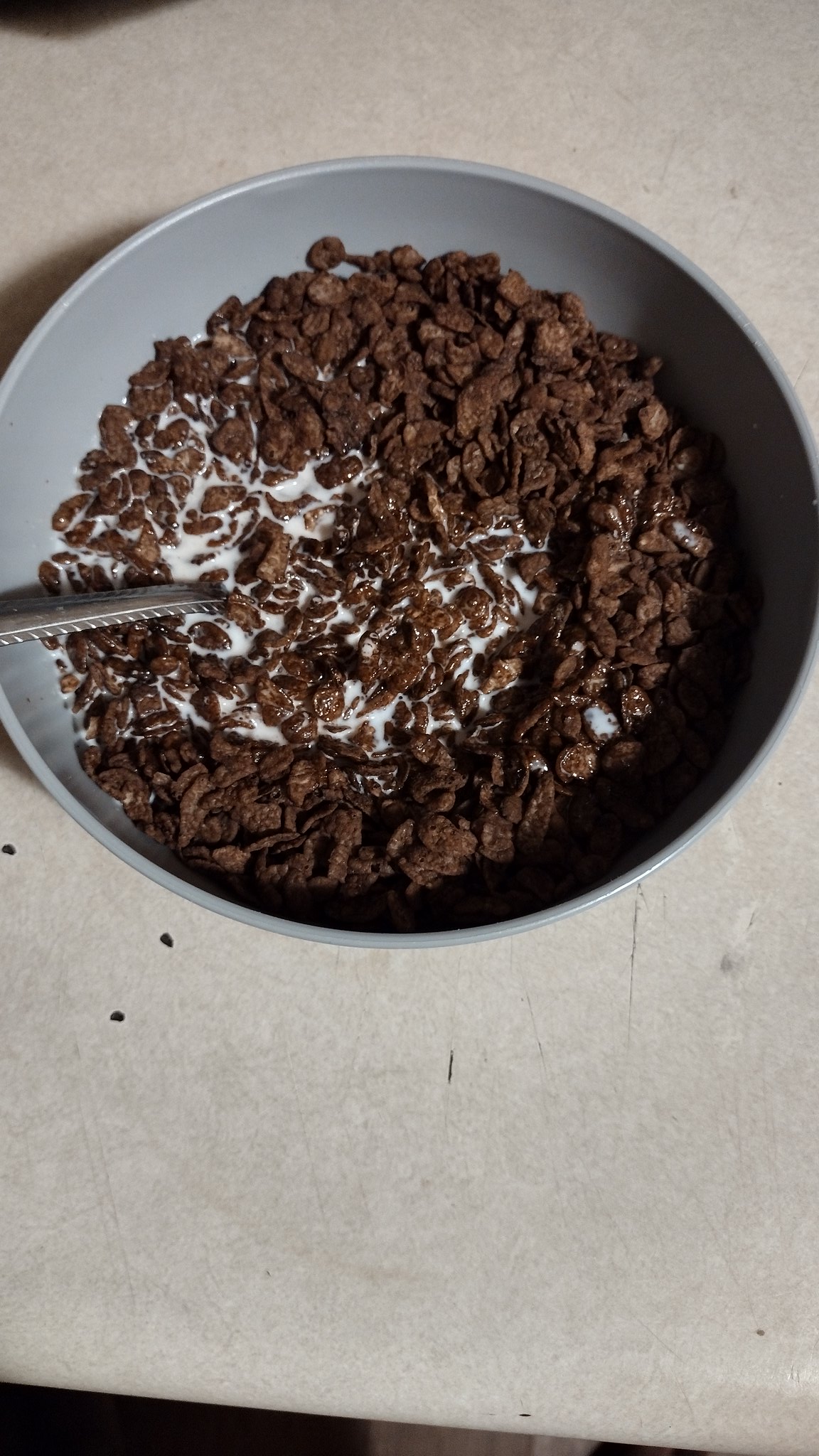The image features a gray bowl filled with what appears to be Cocoa Puffs cereal, sitting on an aged, white laminate table. The table shows signs of wear, with peeling and cracked spots, along with some black scuff marks and dots. Inside the bowl, the chocolate cereal is partially submerged in milk, with more cereal visible to the left and more milk exposed to the right side. A metal spoon, resting inside the bowl, reveals only its handle. The bowl casts a shadow along its left side and behind it, adding to the scene's depth.